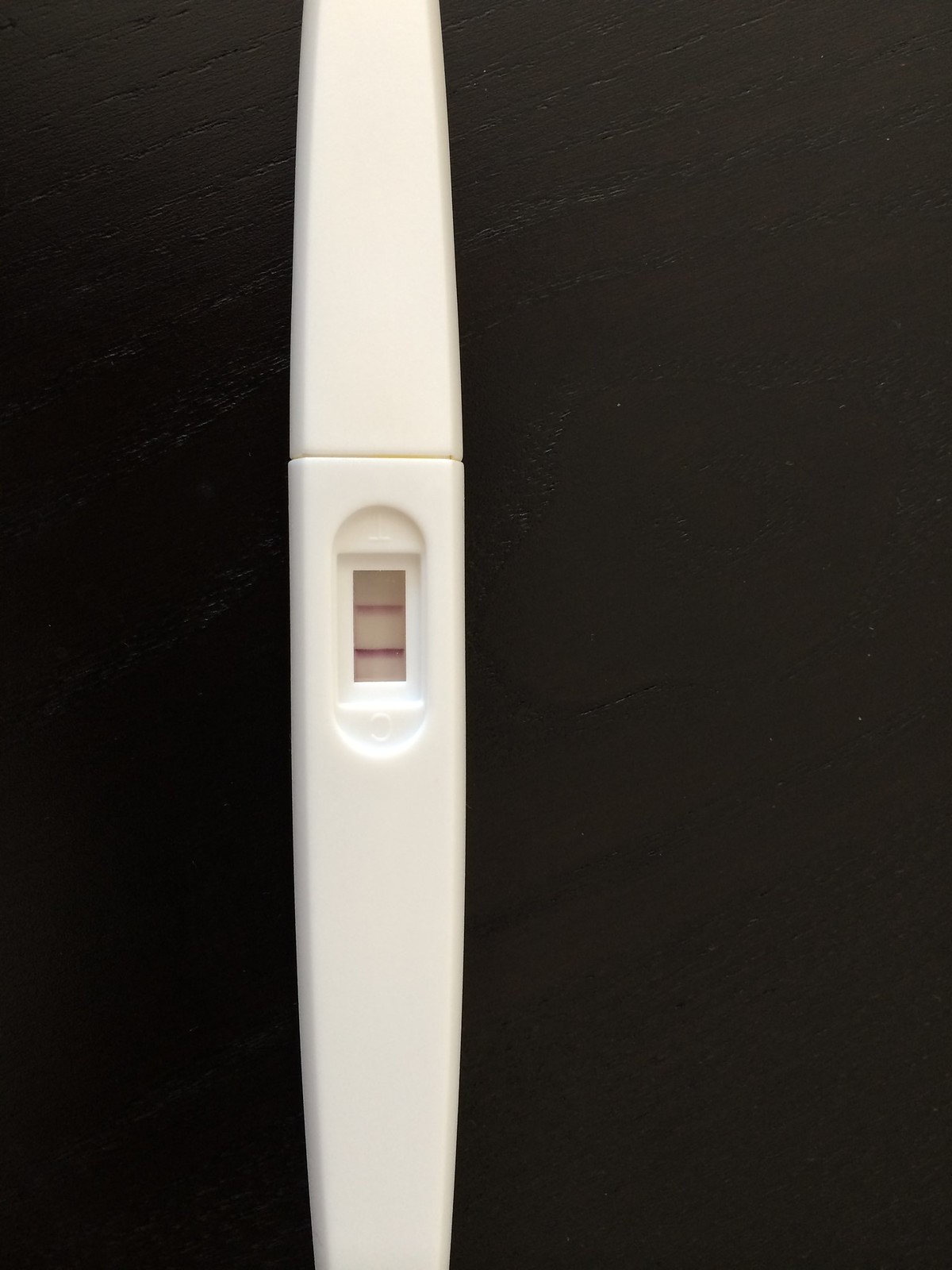Close-up of a white plastic pen-like object placed on a black wooden table. This object, resembling a pregnancy test, features several distinctive details. On its elongated side, there is an indented, capsule-shaped area. Within this capsule-shaped indent is a further recessed rectangle with a clear window displaying two red lines. The top line is a lighter red, while the bottom line appears darker and more pronounced. Above this rectangular indent, the rounded ends of the capsule shape are marked with a "+" symbol at the top and a circle at the bottom. The pen-like object has a cap on one end and a tapered tip on the other, designed for use. The overall appearance suggests it is a pregnancy indicator, intended for use by removing the cap, applying a urine sample, and detecting pregnancy probability based on the test result.